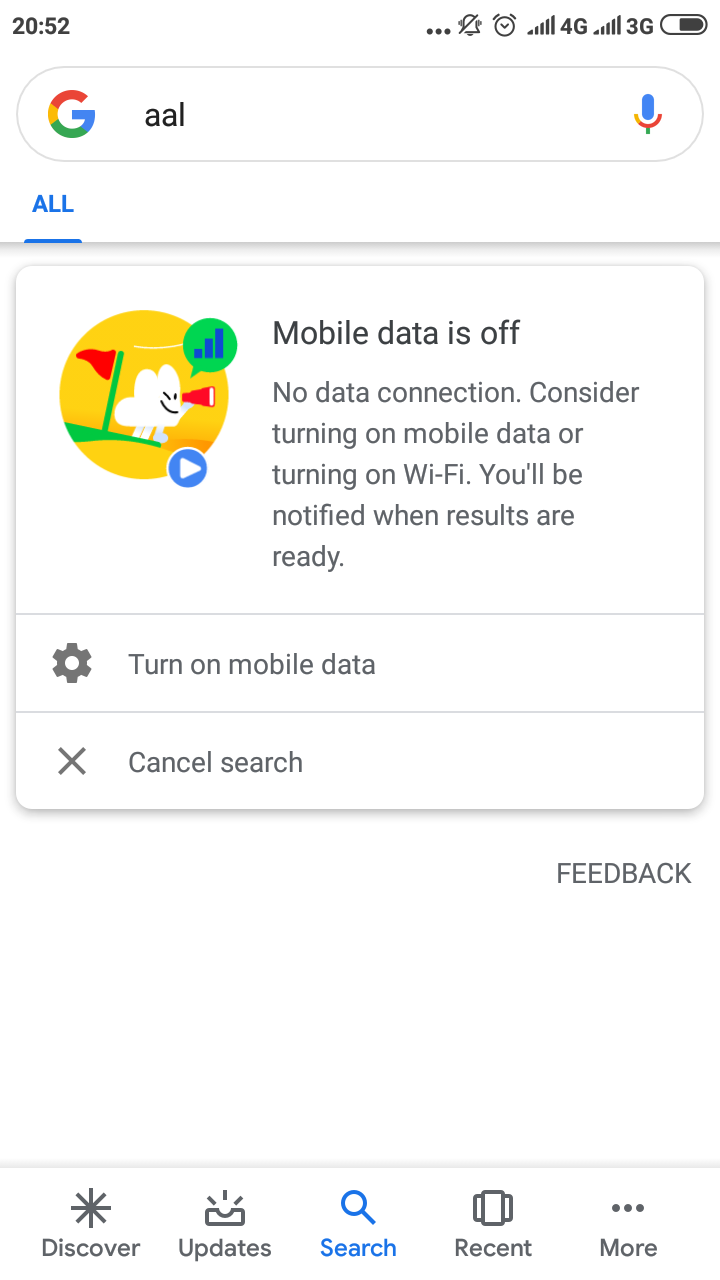A detailed screenshot of a Google search for "AAL," likely taken on an Android smartphone. The screenshot shows the device's status bar at the top, displaying various icons and information. On the far left, the time is shown as 20:52, indicating the use of a 24-hour clock system. On the upper right-hand corner, a row of indicators is present, starting with an ellipsis icon that suggests there are additional notifications not currently visible.

Following this, several symbols are visible: a vibration icon indicating the phone is on silent mode, an alarm clock emblem signifying an alarm is set, and both 4G and 3G data icons, which may indicate the use of a dual SIM smartphone or an active 4G connection with 3G as a fallback. The data signals appear to be at full strength. The battery icon shows an unconventional design where the depletion progresses from right to left instead of the typical left to right, and the battery level seems to be around 25% or 75%.